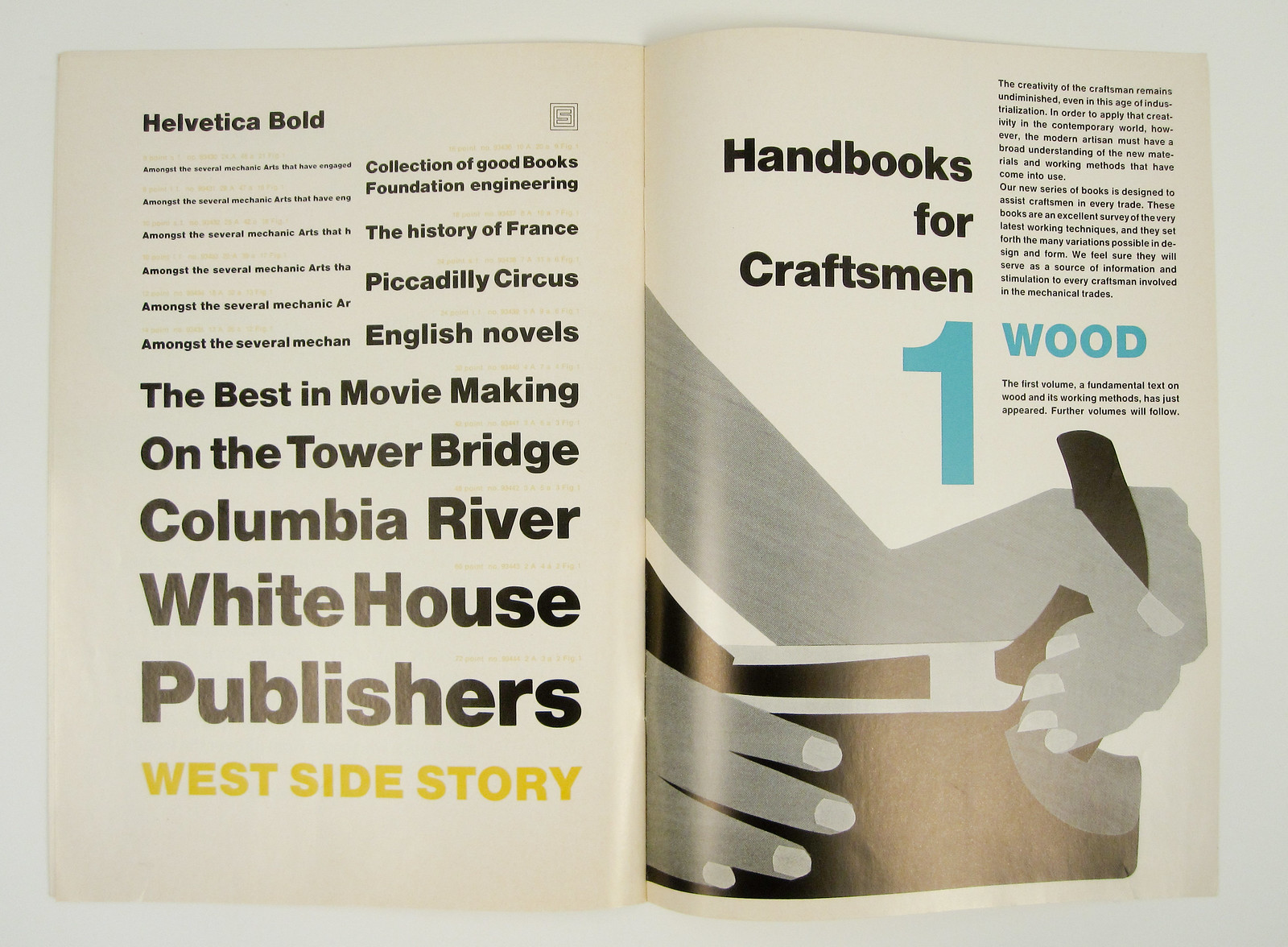The image features a white booklet with progressively larger text on the left side, listing titles such as "Helvetica Bold," "Collection of Good Books," "Foundation Engineering," "The History of France," "Piccadilly Circus," "English Novels," "Best in Movie Making," "On the Tower Bridge," "Columbia River," and "White House Publishers." Positioned underneath these titles, the phrase "West Side Story" stands out in yellow font. On the right side, there is additional text, starting with "Handbook for Craftsmen," and highlighting "One, Wood" in light blue font with more text following. The visual includes a detailed illustration of a craftsman at work, showing two hands grasping an intricate piece of wood, suggesting the individual is engaged in carving a banister or similar wooden object. The person is equipped with a tool belt, emphasizing the theme of woodworking and craftsmanship.